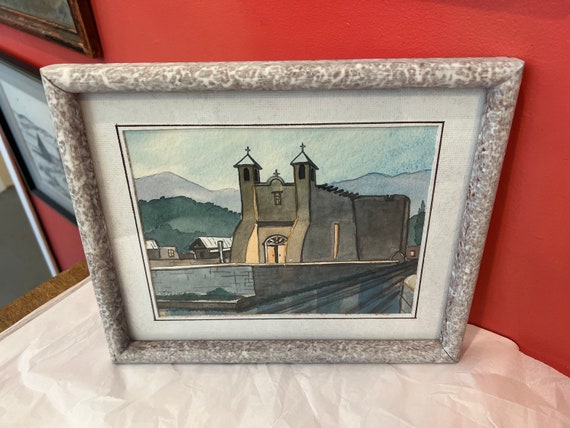This photograph captures a framed artwork with a detailed, watercolor-esque print. The frame, with a border resembling marbled stone in shades of light brown, white, and off-white, encloses an illustration that appears to be of a church. The church features multiple crosses and unique architectural elements such as curved outcroppings and wooden logs reminiscent of Pueblo Indian styles, giving the impression of a structure made from stucco or stone. Accompanying the church are adjacent buildings that resemble barns or structures from a small town. The background of the painting displays distant mountains under a partially blue sky. The framed artwork is positioned on a white-covered tabletop, leaning against a red wall adorned with other photographs and artwork. This setting suggests a museum or an art studio environment.